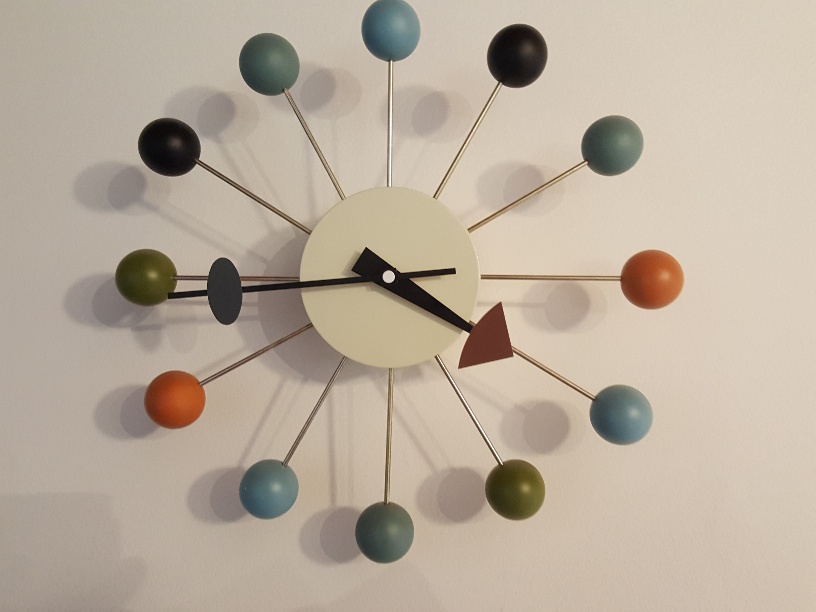In this image, a fun and colorful clock is mounted on a very pale off-white or pale lavender wall with a clear shadow cast to the bottom left. The clock’s centerpiece is a small, white disc with two hands: the hour hand is black with a rust-colored triangular arrow at its tip, and the minute hand features an oblong black shape near its end. Instead of traditional numbers, the clock features twelve silver spikes radiating from the center, each ending in a round ball. These balls come in various colors, such as gray, slate blue, black, reddish-orange, olive green, and purple, giving the clock a lively, eclectic appearance. The time displayed is approximately 4:43 or 4:44. There are no other objects in the background, highlighting the clock’s unique design.